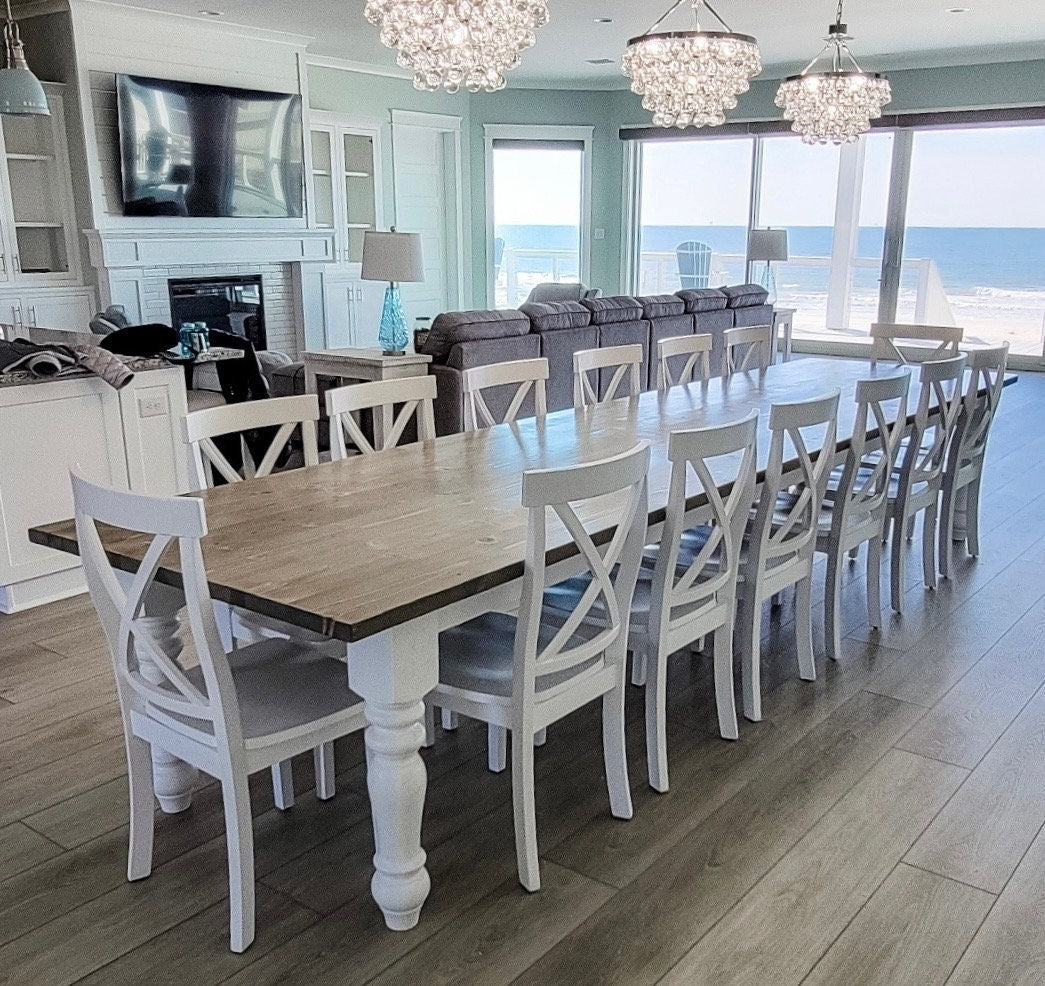The full-color indoor photograph captures a luxurious and expansive dining room bathed in a mix of natural and artificial light during the day. Central to the image is a long wooden dining table, its white legs and brown tabletop anchoring the space with sophistication. The table is flanked by twelve white wooden chairs, six on each side, and two additional chairs at each head, capable of seating 14 people. Above the table hang three ornate crystal chandeliers, casting an elegant glow onto the room.

The floor is crafted from beautiful grayish-brown hardwood, adding warmth and texture. In the upper right corner stands a flat-screen television mounted above a black, unlit fireplace. This area seamlessly transitions into a small living room setup featuring a large sectional couch that could comfortably seat at least six individuals, with a side coffee table adorned by a glass lamp.

The room's colors are a calming palette of whites, grays, and tans. Alongside the top center to the right, large windows and a combination of a modern full glass door and a three-panel sliding glass door reveal a stunning beach vista, complete with sand and the ocean, emphasizing the serene beachfront location of this home. Such a setting would indeed make a dream coastal residence.